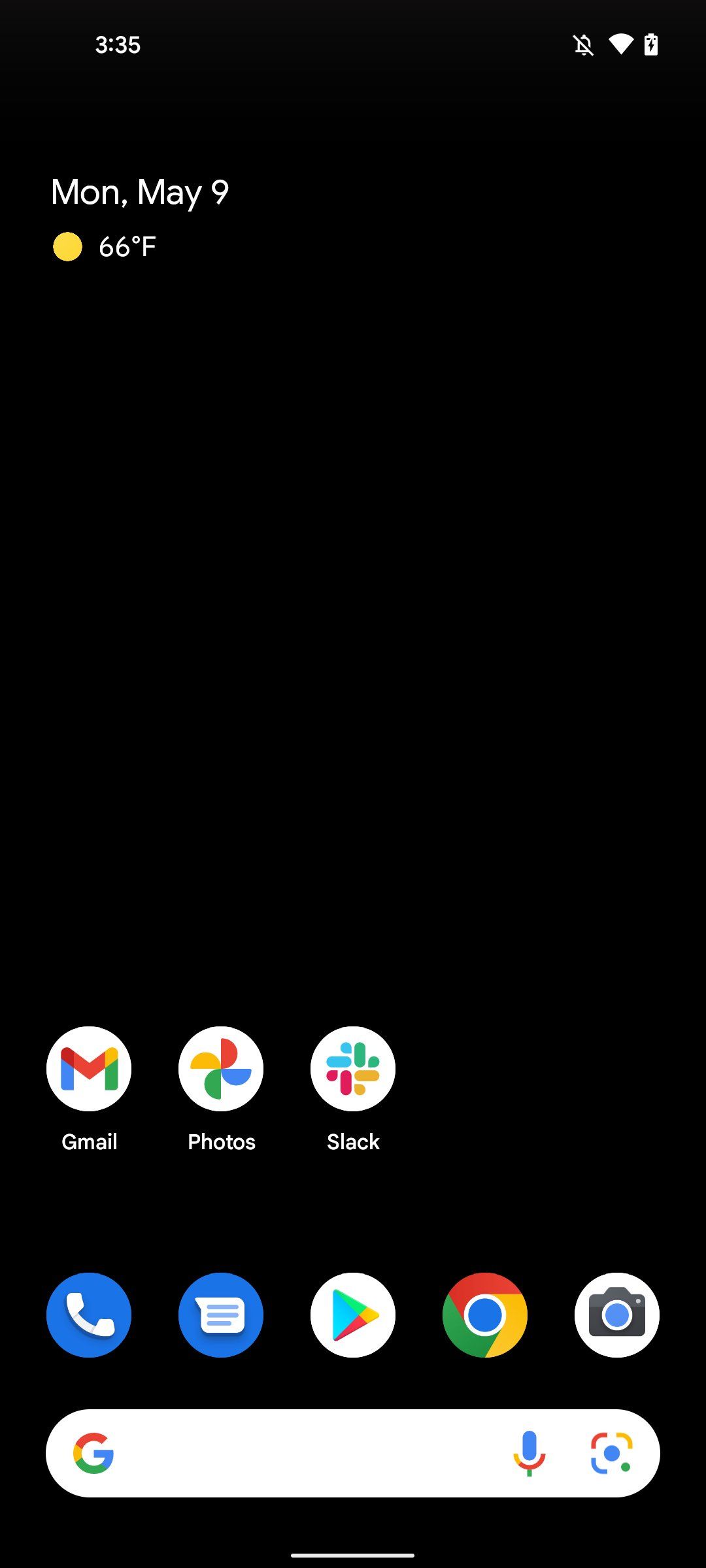This is a highly detailed and organized caption for the image described:

---

The image showcases a phone screen captured at 3:35, presumably a.m. given the pitch-black background. In the upper left corner, "3:35" is displayed prominently. There are no active notifications. The Wi-Fi signal is shown to be strong, but the battery icon indicates it is nearly depleted. 

The date reads "Monday, May 9th," and the weather forecast beside it features a sun symbol with a temperature of 66 degrees Fahrenheit, suggesting sunny weather. 

Occupying the bottom third of the screen are various app icons, neatly arranged in a grid format typical of a Google interface. The top row includes icons for Gmail, Photos, and Slack. The subsequent row consists of icons for Phone, Messages, Google Play Store, Google Chrome, Camera, and a Google search bar.

The simplicity of the black background highlights the app icons, which appear vibrant and organized against the dark canvas.

---

This caption organizes the information into a coherent, reader-friendly format, emphasizing key details while maintaining clarity and descriptive depth.